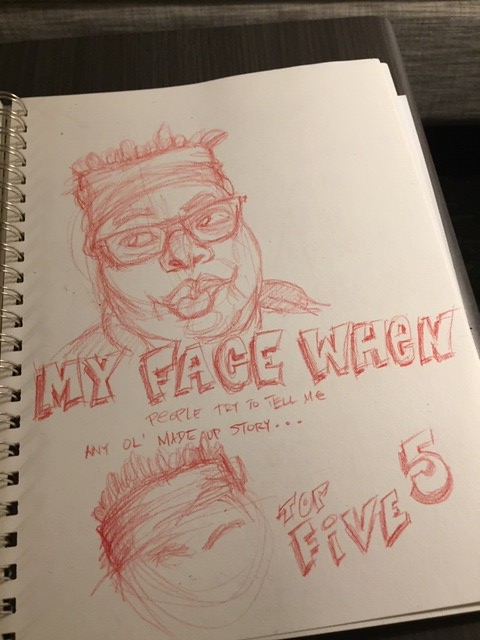In this vertical, rectangular image, an open artist's sketchbook with spiral binding is prominently displayed against a dark brown desk or tabletop. The cream-colored paper of the sketchbook contrasts with the intense red hues of the drawing. The visible page features a detailed sketch of a woman wearing a headband. She has dark-rimmed glasses, full lips, and her shoulders and part of a collar are visible. Above the portrait, block text in the same red pencil reads: "My face, whew, people try to tell me my old made-up story. Any old made-up story, top five." The combination of text and illustration creates a compelling visual narrative, capturing the viewer's attention with its bold, monochromatic scheme.